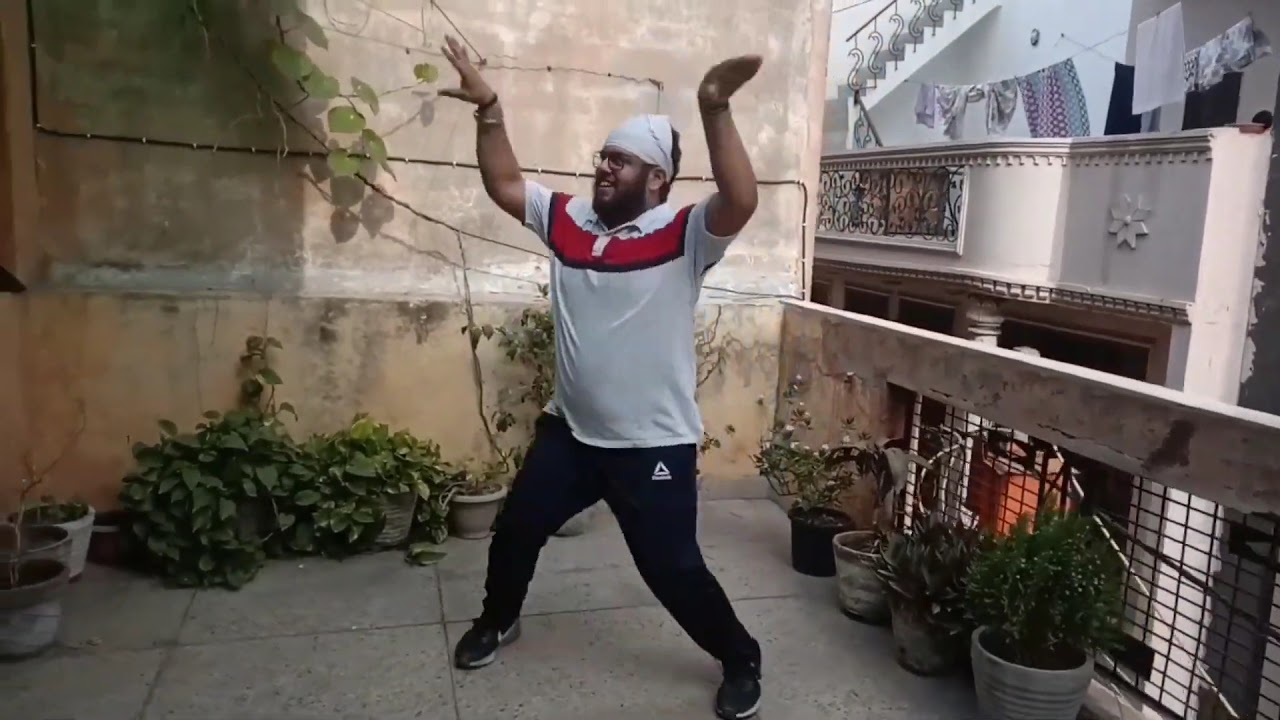The photograph captures a joyous moment as a man dances exuberantly on the rooftop of a building. His feet are stretched, knees bent, and arms are raised upwards, bent at the elbows, suggesting movement. He is smiling broadly, and his gaze is directed upwards. The man is dressed in a white t-shirt with red accents near the shoulders, a white cloth resembling a bandana on his forehead, blue pants, and black shoes. He wears spectacles and has a beard.

The rooftop is adorned with potted plants, adding a touch of greenery to the scene. The background features a peach-colored wall, creating a warm contrast. To the right, another building is visible, featuring a balcony with a clothesline hanging with clothes drying, and a staircase is present near the clothesline. A metal railing can be seen, emphasizing that the man is elevated, possibly on a balcony. The adjacent structure hints at additional levels, with a banister visible in the upper right. The scene is set against the backdrop of an interconnected urban environment, capturing a lively and joyful rooftop moment.